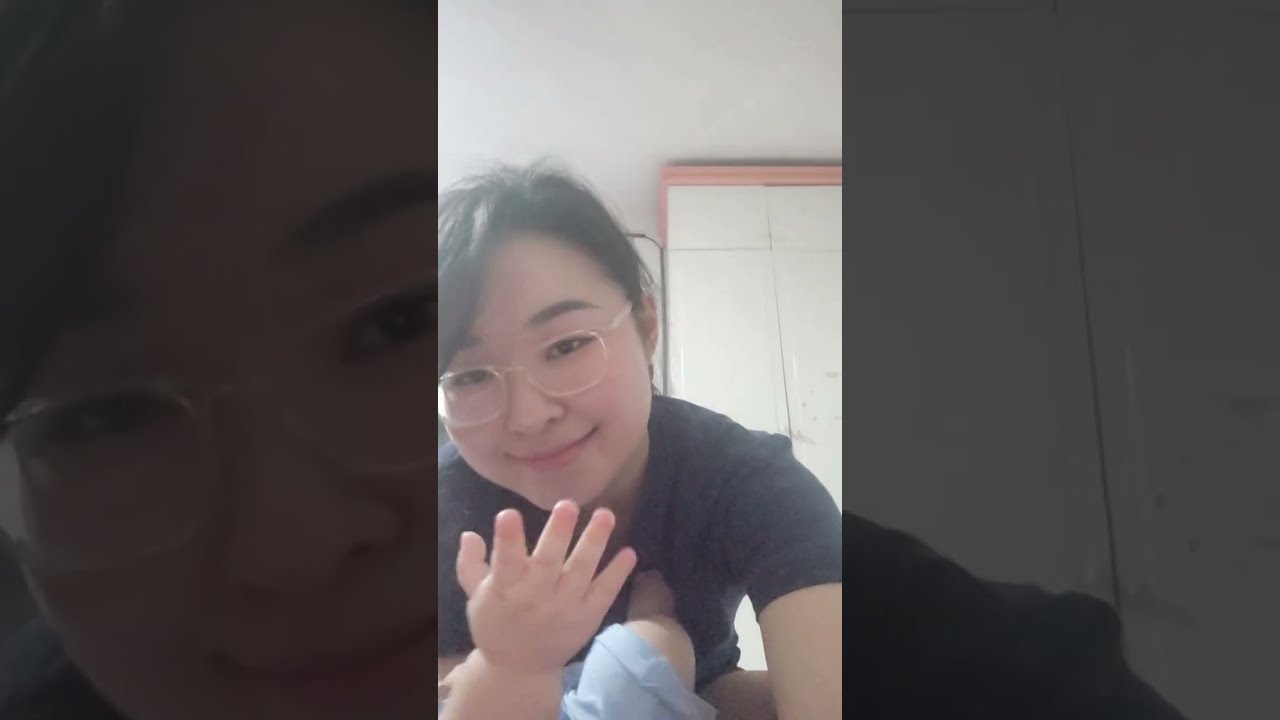In this photograph, we see a woman of Asian descent smiling at the camera, likely taking a selfie. She has dark hair pulled back into either a ponytail or a bun, with bangs swooping to the side. She is wearing clear or pink eyeglasses and a black short-sleeve t-shirt. Her dark hair is parted to the left side, complementing her thick black eyebrows. She has noticeable red lips, adding a pop of color to her look.

In front of her, there is a baby or toddler, dressed in a light blue outfit or blue shorts, with their leg pressed against her chest and their hand visible in front of her face, emphasizing the close bond between them. The background features a white wall with red trim at the top and a white ceiling. On the right side of the image, a large shelf with white doors is partially visible. The overall composition captures a tender and joyful moment between the woman and her child.